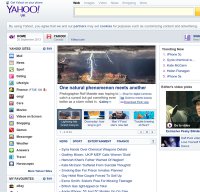This screenshot showcases a Yahoo homepage from at least 20 years ago. Prominently featured on the top left is the classic purple Yahoo logo, complete with its iconic exclamation mark. Adjacent to the logo on the right, there is a search bar and address bar for user queries. Below the search bar, the left-hand side displays a series of approximately 10 to 15 navigational tabs, likely corresponding to categories like movies, music, and sports, though the small, blurry quality of the image makes the exact labels indiscernible. 

In the center of the page is a headline image capturing a dramatic lightning strike in what appears to be a desert landscape, though the accompanying text is too unclear to read. Beneath this main image, there are four additional thumbnails, presumably linking to other articles. The background of the webpage is a stark white, contributing to the overall minimalistic and subdued color scheme of the screenshot.